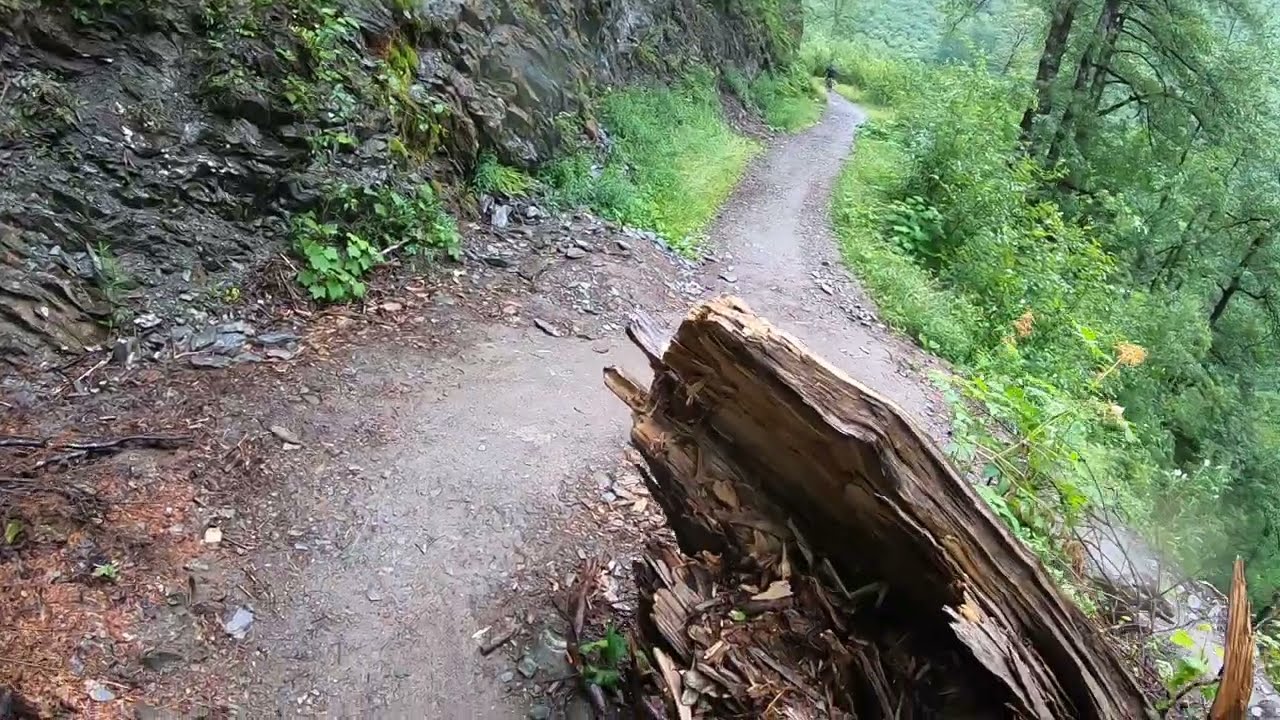The image depicts a dirt path running centrally through a wooded area, viewed from a slightly higher vantage point. The path is well-worn, slightly slick, and appears damp, suggesting recent rain or morning dew. It winds through a densely vegetated forest, with a rock wall on the left, covered sparsely with moss and vegetation, hinting at an uphill terrain or cliff. In contrast, the right side features a drop-off into a lush, green forest adorned with thin tree trunks and a few light orange or golden flowers. Prominently in the foreground, a decomposing log stretches from the center towards the right, possibly causing the path to split around it. The lower left quadrant shows smaller rocks and an open space of medium gray dirt or pavement with scattered dried leaves. The entire scene is encapsulated within a wide rectangular frame, providing a detailed glimpse into this serene woodland trail.